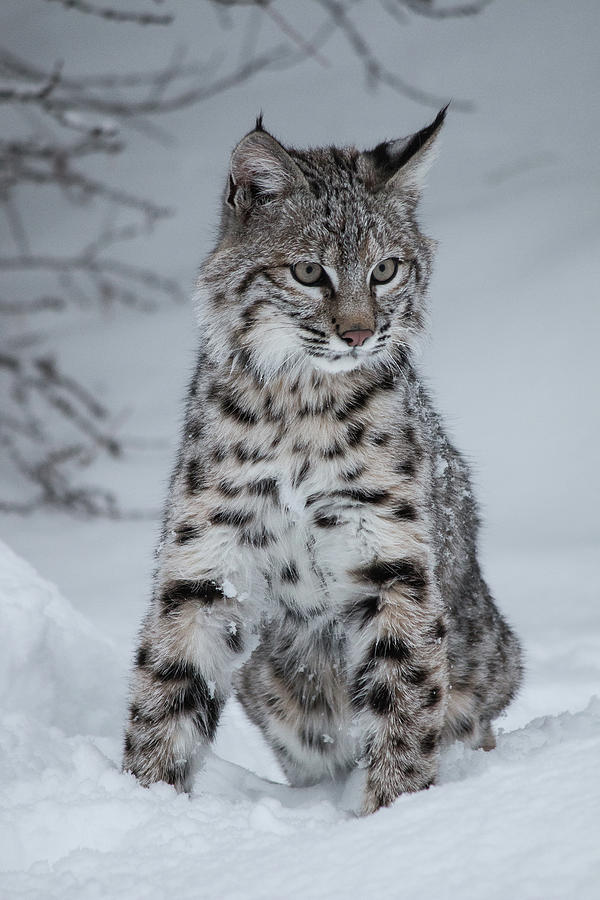In this captivating color photograph, a bobcat or lynx is elegantly poised in a snowy, woodland setting. The majestic wildcat sits on its hind legs with its front legs straightened, its feet partially buried in the fluffy snow that blankets the landscape. The lynx, part of the wildcat family, features pointed ears adorned with tufts of black hair, a distinguishing characteristic of its species. Its coat showcases a mesmerizing blend of gray, white, beige, and brown, adorned with black spots. 

The lynx's face is marked by expressive green eyes with black pupils, a pink nose, and a white snout accentuated by black stripes. It gazes slightly to its left, seemingly focused on something in the distance. Surrounding the bobcat, bare trees and leafless branches rise from the snow-covered ground, indicating the frigid climate. The intricate details of the bobcat's appearance and the serene, frozen environment capture the raw beauty of nature in this stunning image.